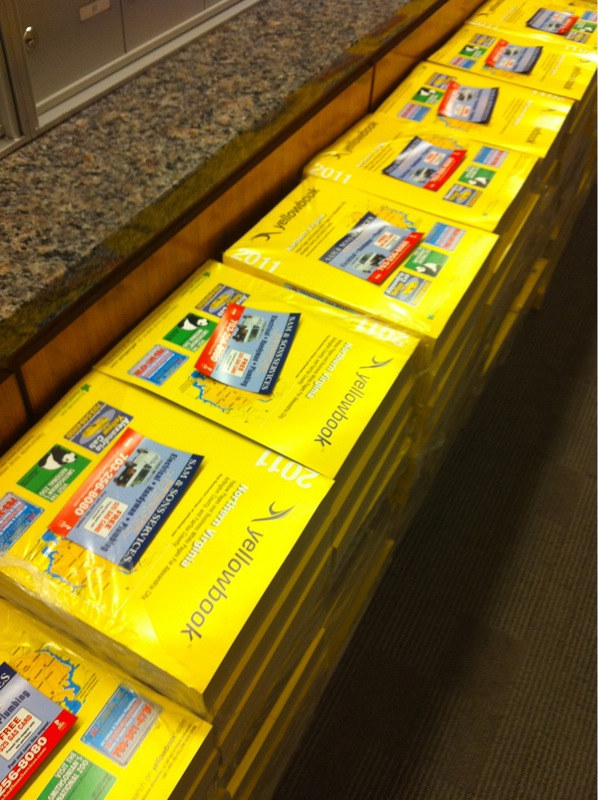The image depicts a cluttered array of thick, yellow phone books, commonly known as Yellow Pages, stacked approximately a meter high and shrink-wrapped in plastic. These outdated directories, bearing the year 2011 on their covers, form a 'wall' situated against a low, wooden partition. Adjacent to this partition is a metal wall with a narrow strip of either marble or granite, smooth in texture with beige, brown, and black markings. A notable feature above the stacks is a series of small, silver mailboxes, each equipped with a lock, suggesting that this area serves as the building's mailroom. The floor in front of the stacked books is covered with dark grey carpet tiles adorned with thin, light grey stripes, adding to the somewhat dated ambiance of the scene. This snapshot captures the relic status of these Yellow Pages, waiting in a common area for potential retrieval.